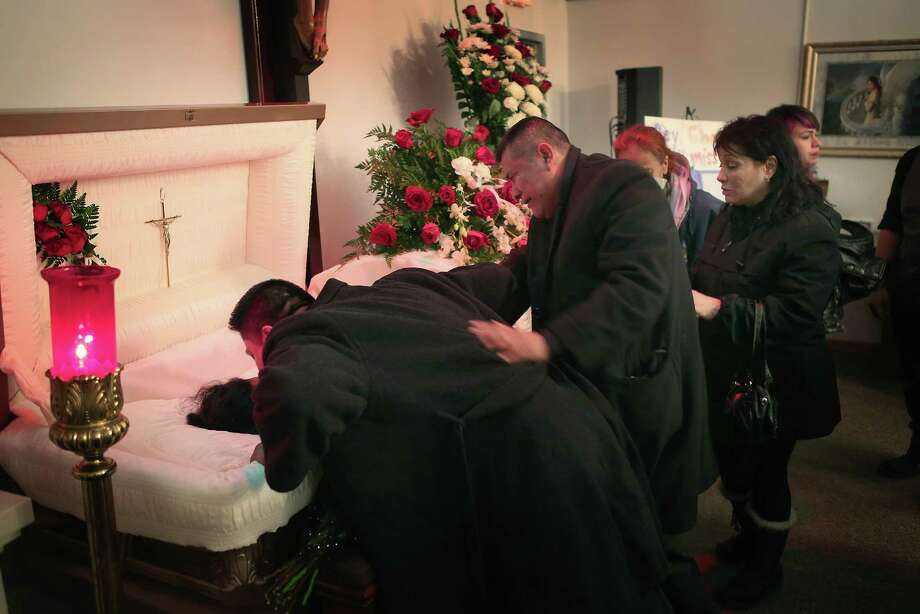The photograph captures a solemn scene from a Christian funeral wake. The focal point is an open casket positioned on the left side of the image, adorned with a crucifix on the inner lid and lined with pristine white fabric. A deceased individual lies peacefully inside. Surrounding the casket, four people—two men and two women—are dressed in black as a mark of respect. The men are kneeling, with one visibly bent over either speaking to or kissing the deceased, while a woman third from the front wears distinctive snow boots with white fluffy tops. The emotional weight of the moment is palpable, with one of the men appearing to cry. A pink-glassed candle holder sits in the foreground to the left, casting a warm light. The setting is enriched by red and white flowers with green leaves, and pictures with gold frames hanging on the wall to the right. The background shows no text, but the scene is vividly colored with hues of white, red, pink, yellow, green, black, and gray, likely within a church. The gray floor underscores the mournful ambiance of this final farewell.